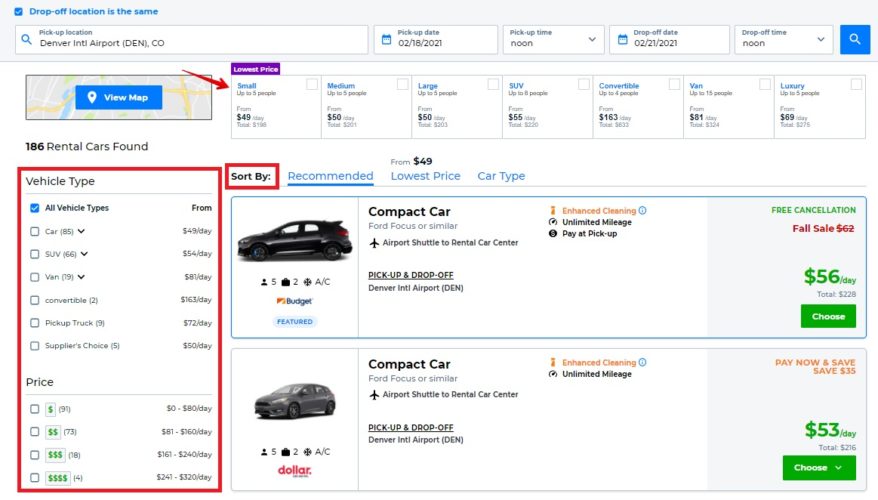The image is a screenshot of a car rental website displaying search results for rental cars. In the upper left corner, the search box shows a query for vehicles to be picked up at Denver International Airport (DENCO) on February 18, 2021, at noon, with a return set for February 21, 2021, also at noon. The left side of the screen shows a highlighted section denoted by a red square, drawing attention to the vehicle type filters. Additionally, a smaller red triangle focuses on the "SORT BY" option to the right. Above the "SORT BY" label, a red arrow points to the "Lowest Prices" section, which indicates the most affordable option available, listed at $49.